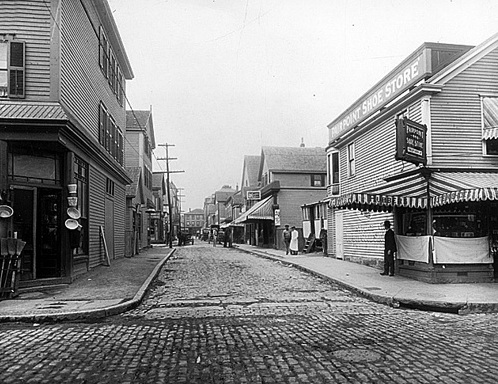This black-and-white photograph captures a bustling, cobblestone street scene at a multi-way intersection, possibly a three-way or four-way junction. The street is composed of individually laid cobblestones, adding an old-world charm to the image. The camera is angled down one of the streets, with houses lining both sides.

Dominating the right side of the photo is a two-story building prominently displaying the "Four-Point Shoe Store" sign in white letters, both above the entrance and extending from the side of the building. The store features striped awnings on both corners, providing shade beneath which a gentleman stands. Further along the sidewalks, other pedestrians can be seen strolling, dressed in what appear to be dresses and suits, though the distance makes precise details unclear.

Opposite the shoe store, another two-story building with a corner entrance stands, contributing to the urban feel of the scene. A utility pole is visible on one side of the street, while the sky, appearing light gray in this black-and-white format, looms overhead, setting a reflective tone for the photograph.